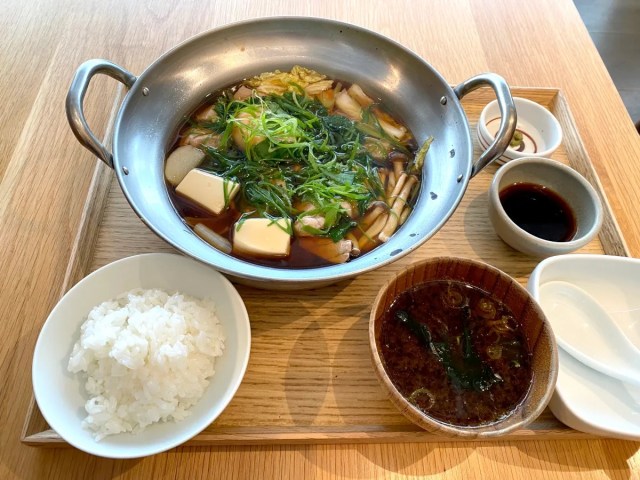The photograph depicts a meticulously arranged meal on a light wood tray, set upon a slightly darker wooden table. The central focus is a round, metal pot with handles, containing a savory Asian soup featuring long white mushrooms with brown tops, cubes of tofu, and a variety of vegetables including what appears to be cabbage or daikon. The soup is garnished with green onions and sits in a dark broth. Surrounding the pot on the tray are various components that complete the meal. In front and to the right of the pot is a white bowl filled with fluffy white rice, and beside it is a darker, wooden bowl holding a rich, dark-colored liquid, possibly another type of soup. A rectangular plate with rounded edges holds a Chinese-style soup spoon, and behind it, there's a gray bowl likely containing a dipping sauce, perhaps soy sauce. Adjacent to these items is a white ramekin with a dark sauce and another bowl featuring a red spiral pattern on its interior, creating a visually appealing spread that highlights both the diversity and harmony of the meal.